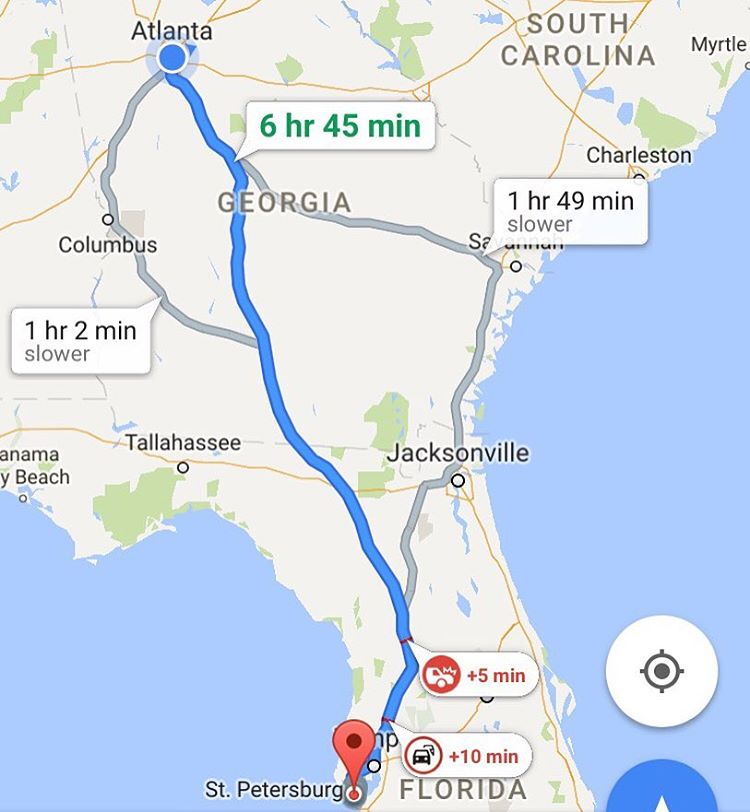The image is a detailed screenshot from Google Maps, depicting a car route through the southeastern United States. The map showcases parts of South Carolina, Georgia, and Florida, with a focus on a journey from Atlanta, Georgia, down to St. Petersburg, Florida. This primary route is highlighted with a blue line and indicates a travel time of six hours and 45 minutes, displayed prominently in green ink within a white banner. The destination, St. Petersburg, is marked with a red icon on the coast of Florida.

Additionally, the map features two alternative routes in gray. The left alternate route, which reroutes through Columbus, Georgia, is marked with a flag indicating it is one hour and two minutes slower. The right alternate route runs through Savannah, Georgia, and Jacksonville, Florida, and is marked as one hour and 49 minutes slower.

Several points of interest and warnings are included on the blue route. Notably, two red lines signify areas of concern. The first red line, which includes a red circle with a white car icon indicating a crash, notes a delay of five minutes. Further south, close to the destination, another red line bears an icon showing two cars, suggesting a ten-minute delay due to extra traffic.

The map also contains textual elements and markers: Atlanta is denoted with black text and a blue dot, while St. Petersburg is marked with an orange pin and its name in black text. At the bottom right of the image, there are two circular icons – a white one and a blue one with an arrow pointing upwards.